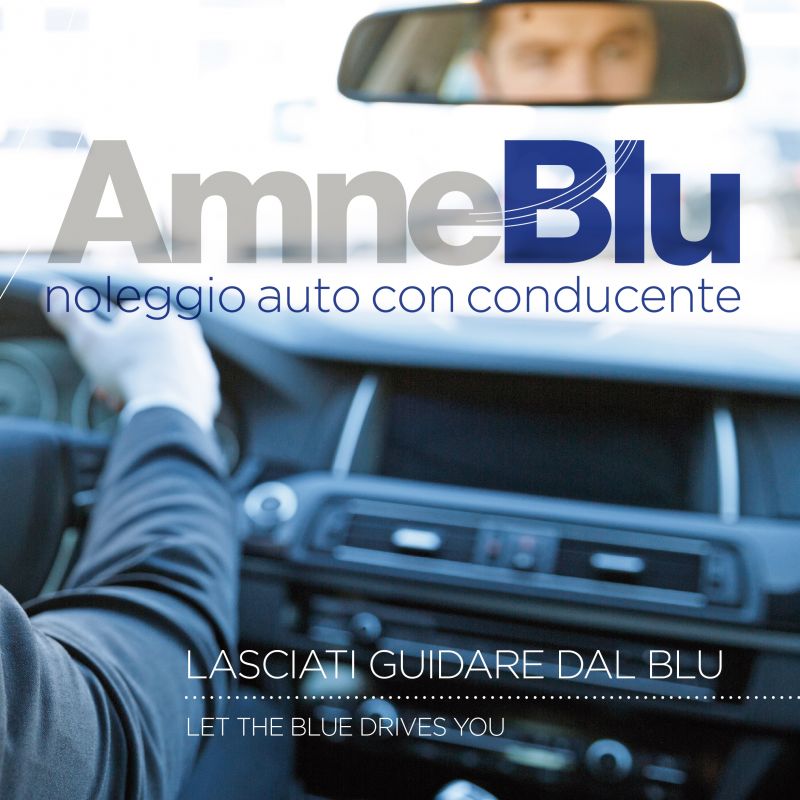The photograph captures the interior of a car's dashboard, specifically on the right side of the steering wheel where a hand grips it. The hand belongs to a person whose partial reflection—showing their forehead, eyes, and part of the nose—is visible in the rearview mirror mounted at the top of the image. Their light-colored skin contrasts with a dark top or suit. 

To the right of the hand, various controls for the air conditioning and stereo system are visible. The world outside the car is bright and hazy, adding an indistinct, white backdrop. 

Overlaying the image, the text "AMNE" is displayed in gray across the bright windshield, followed by "BLU" in a darker navy blue. Below this, in thin white text against the dashboard, it reads "noleggio auto con conducente" (Italian for "car rental with driver"), followed by a dotted line and the English translation, "Let the blue drive you." This composition suggests the photograph is part of an advertisement, possibly for a rental car service or insurance, emphasizing the ease and tranquility of using the service on a sunny day.